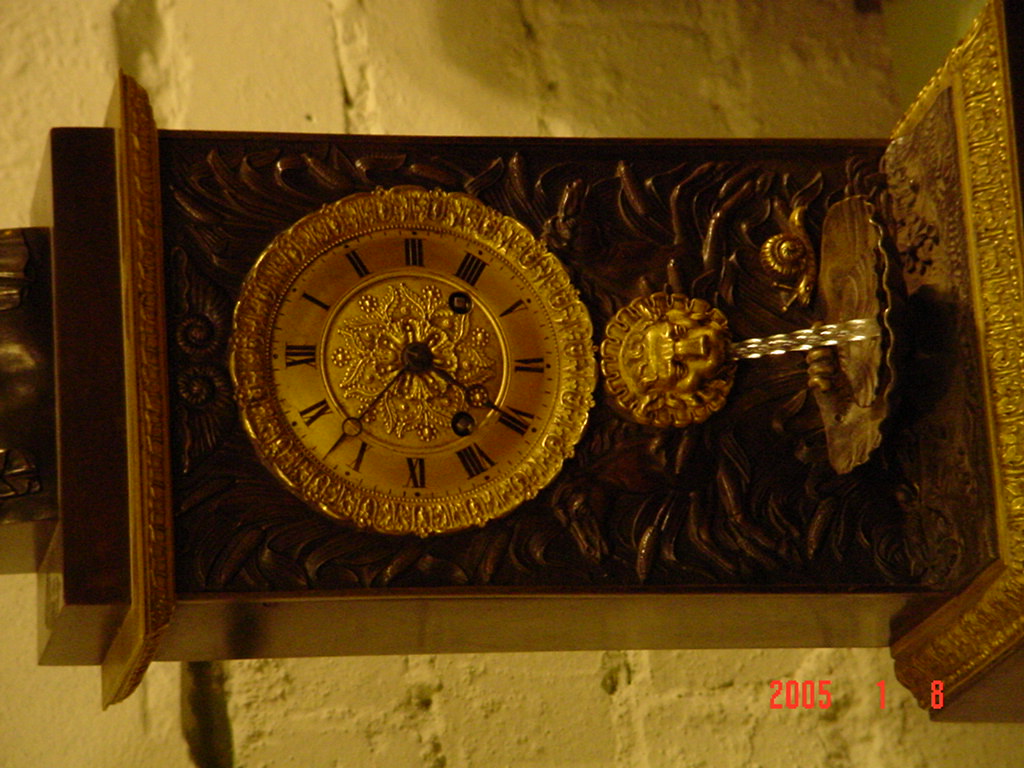This photograph captures an exquisite antique clock with intricate details, taken on January 8, 2005, as indicated by the red datestamp at the bottom of the image, reminiscent of older camera prints. The clock, predominantly a goldish-bronze hue, is depicted horizontally despite being designed to stand upright. The ornate clock face is adorned with delicate floral engravings behind the hands, adding to its elegant appearance. Below the clock face, a lion’s visage intricately sculpted appears to be a decorative fountain, with water seemingly spouting into a small basin resembling a soap dish. The entire structure is rich with lavish embellishments, embodying a sense of timeless sophistication. This smaller, opulent clock looks ideally suited for display on a polished table.